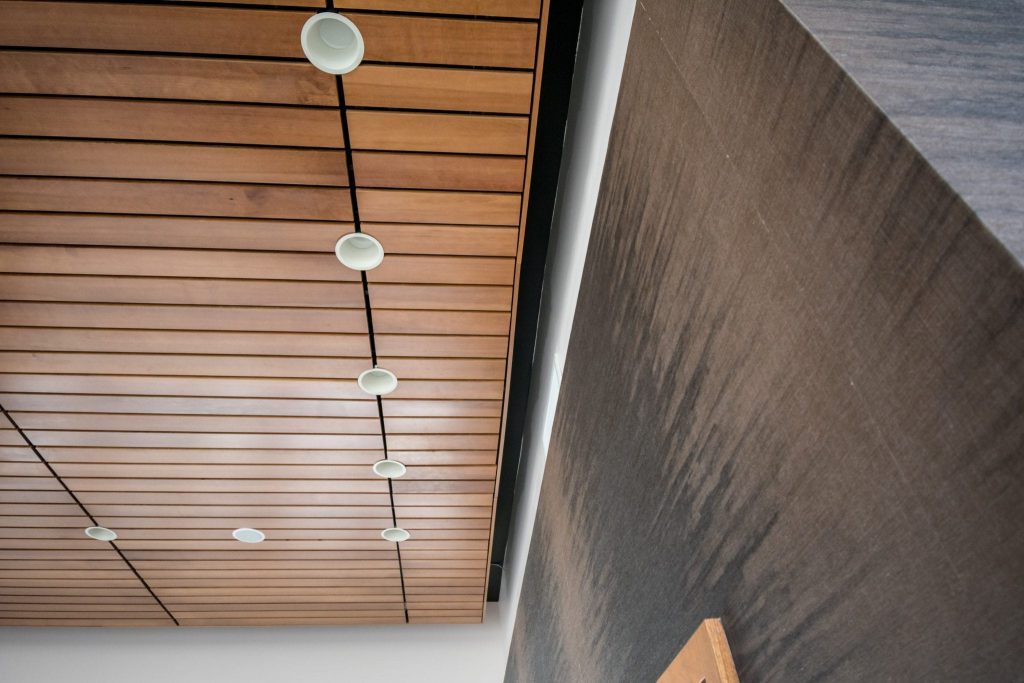This photo, which appears to be taken from an unusual, possibly upside-down, angle inside a modern restaurant, showcases a striking ceiling and wall design. The slatted wooden ceiling, characterized by pale wood slats with black lines between them, features recessed white lighting arranged in white circular fixtures. On the right side of the image, there is a large wall made of polished light gray stone, notable for its shiny finish. Just below this gray wall, a portion of a light brown chair or bench is visible, leaning against the wall. The image also reveals that both the ceiling and the stone wall are bordered by a regular white wall, though this detail is somewhat obscured by the angle. The overall sharp, clean lines and minimalist design suggest a Japanese influence in this visually intriguing restaurant space.